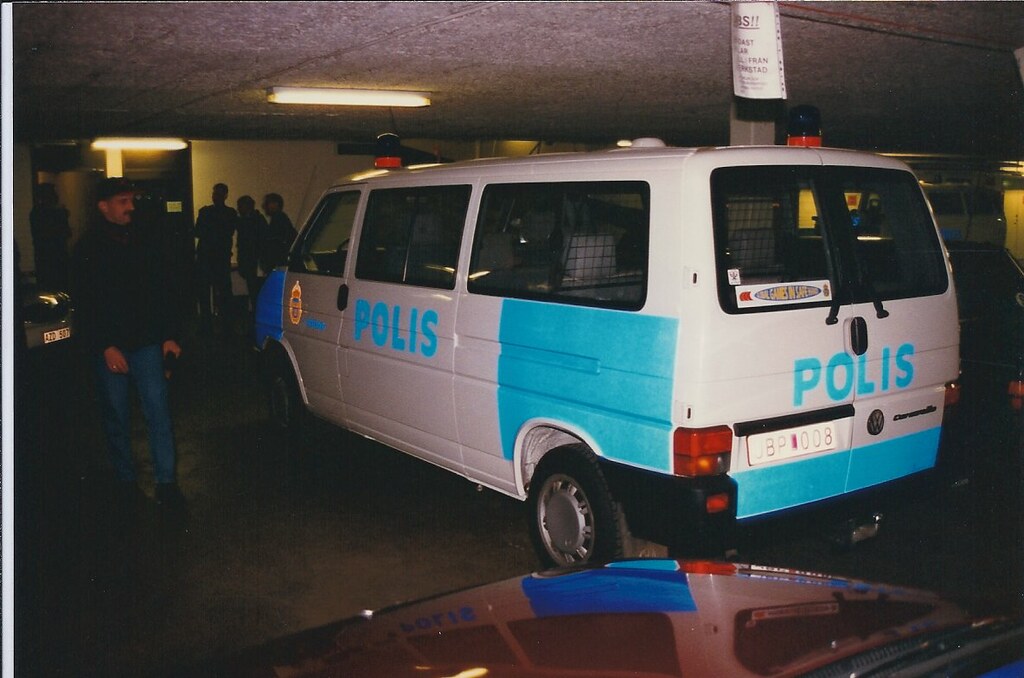The photograph depicts an indoor parking garage with a low ceiling featuring bright tube lights. Dominating the scene is a white and blue police van, prominently displaying the word "POLIS" in blue lettering on its sides and rear. The van also carries a license plate marked JBP-007 and bears the Volkswagen logo, with sirens on top that are currently switched off. The van is situated very close to the ceiling, emphasizing the limited height of the garage. A red car is partially visible in the bottom right corner of the image.

Surrounding the police van are several people, including a man dressed in jeans and wearing a hat standing to the left, intently observing the vehicle. In the background, near the wall, three other men are also present, contributing to a scene that suggests the presence of police personnel. The context hints at a potentially urgent or official situation unfolding within this enclosed and brightly lit space.